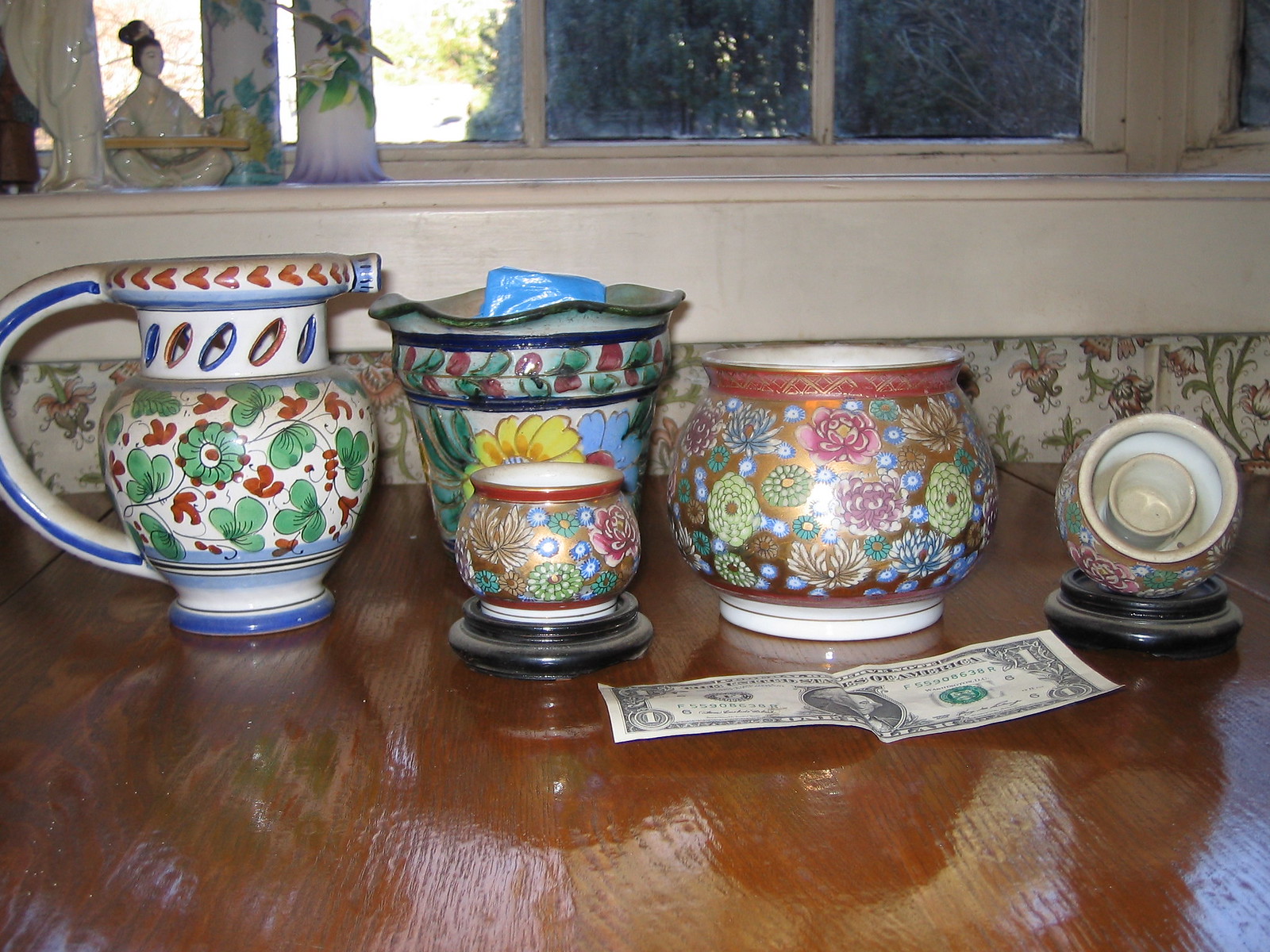The photograph captures a detailed and perhaps cozy scene within someone's home, potentially mistaken for a quaint restaurant. The focal point is a glossy, medium-dark brown wooden table adorned with various ceramic objects and floral-patterned dishware. Above and behind the table, a window framed with ornate floral wallpaper allows light to filter through, enhancing the reflective surface of the table. 

In the upper left corner, a windowsill displays porcelain figures, including a partially visible one and a seated Asian woman figure, possibly Japanese or Chinese, with objects lying across her lap, flanked by two other small figures or candles. The porcelain objects add a touch of cultural intrigue and nostalgic charm to the space.

On the table itself, a dollar bill is unfolded, suggesting a casual or practical household moment. To the left, a white teapot features intricate decorations with green and brown flowers, blue and brown circular patterns, and a blue stripe on the handle. Next to this, another similarly ornate teapot showcases a mix of yellow, blue, and green flowers.

Several ceramic jars and cups of varying shapes and sizes populate the wooden surface. Notably, three larger pieces resemble cups or coffee mugs—all adorned with colorful floral patterns—and two smaller, circular containers, possibly candle holders with dark bases, enhance the table's eclectic vibe. Among the cups, one miniature teacup is noticeably tilted towards the camera, revealing intricate details in its design, adding to the overall visual interest and complexity of the scene.